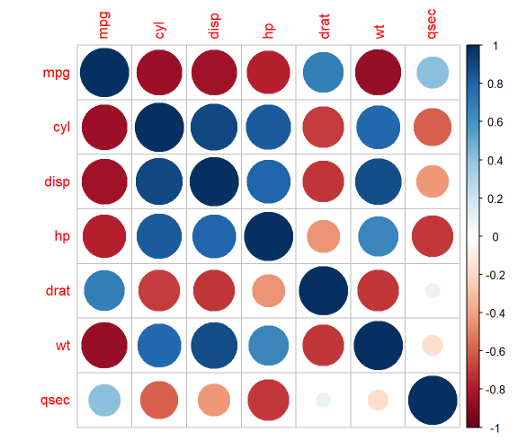The image depicts a detailed heat map and correlation matrix presented in a 7x7 grid. Both the rows and columns are labeled with the same set of variables: MPG, CYL, DISP, HP, DRAT, WT, and QSEC. The matrix is visually represented using circles of varying sizes and colors within each square, indicating the strength and direction of the correlations between these variables. On the right-hand side, a color gradient scale ranges from 1 to -1, with shades of blue representing positive correlations (up to +1) and shades of red representing negative correlations (down to -1), passing through white for zero correlation.

The heat map highlights that when the same variable is compared against itself (both horizontally and vertically aligned), the squares are filled with dark blue circles, indicating perfect positive correlation. Most variables exhibit varying degrees of correlation, with notable exceptions where DRAT and QSEC with MPG show a lack of significant correlation. Additionally, the specific coordinates where DRAT aligns with QSEC (5th row, 7th column), WT aligns with QSEC (6th row, 7th column), and QSEC aligns with both DRAT (7th row, 5th column) and WT (7th row, 6th column) contain no circles, signifying a zero or negligible correlation in these instances. The visualization makes it easy to identify relationships between the variables through the color and size gradients of the circles.